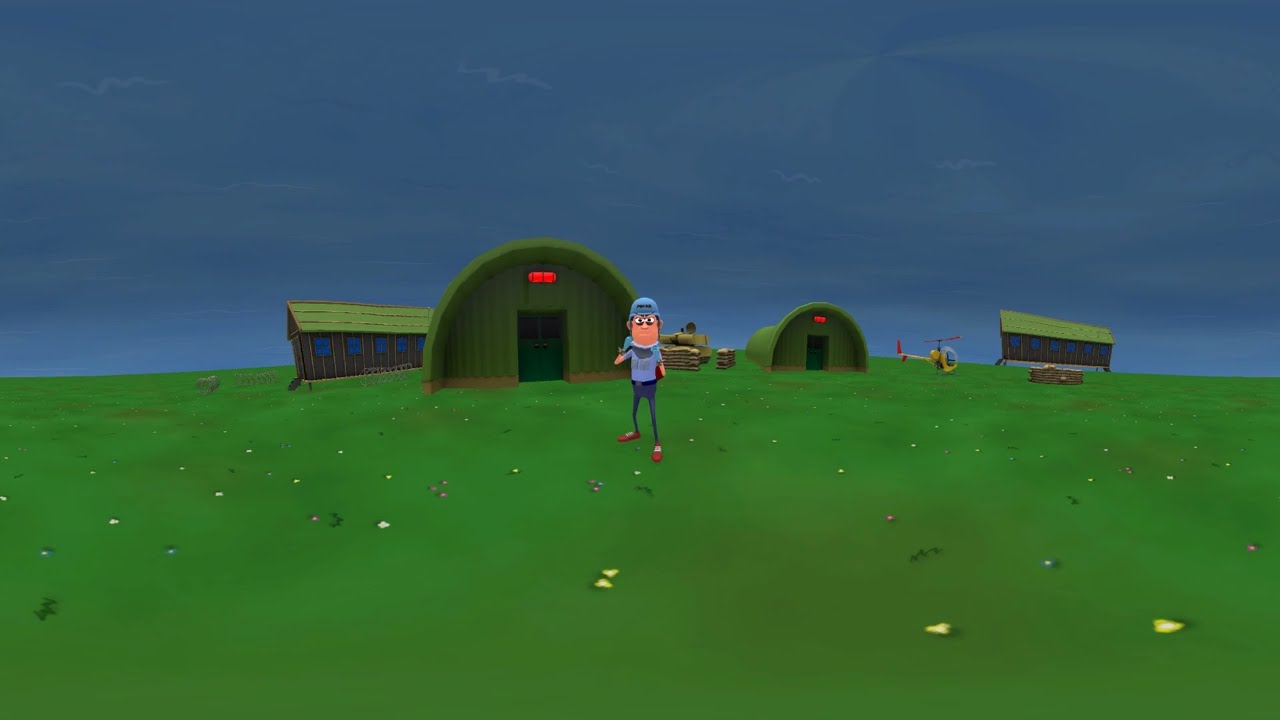This detailed image appears to be a screenshot from a video game or animated video. It is framed by thin black rectangles at the top and bottom, giving it a wide rectangular shape. Dominating the center of the scene is a digitally-created character, a man with a cartoony appearance. He is dressed in a light blue shirt, blue cap, dark blue pants, and red shoes. His one foot is slightly forward, and both small hands are raised to the sides of his chest. His striking features include white eyes set against a green face and pencil-thin legs.

The background features multiple structures. Directly behind the character are large, green, arch-topped buildings resembling airport hangers, each with a red light at the top and an open square door. Further back, there are long brown barns with slanted green roofs and blue windows. On the right side of the image stands a yellow helicopter facing to the right, accented with a red tail.

The ground is mainly a dark green lawn speckled with yellow and dotted with shiny, gem-like objects in purple, pink, yellow, and green. The sky, occupying the upper half of the image, is a deep dark blue adorned with faint white, squiggly lines representing clouds. The overall feeling of the scene is playful and animated, akin to what one might find in a video game world.